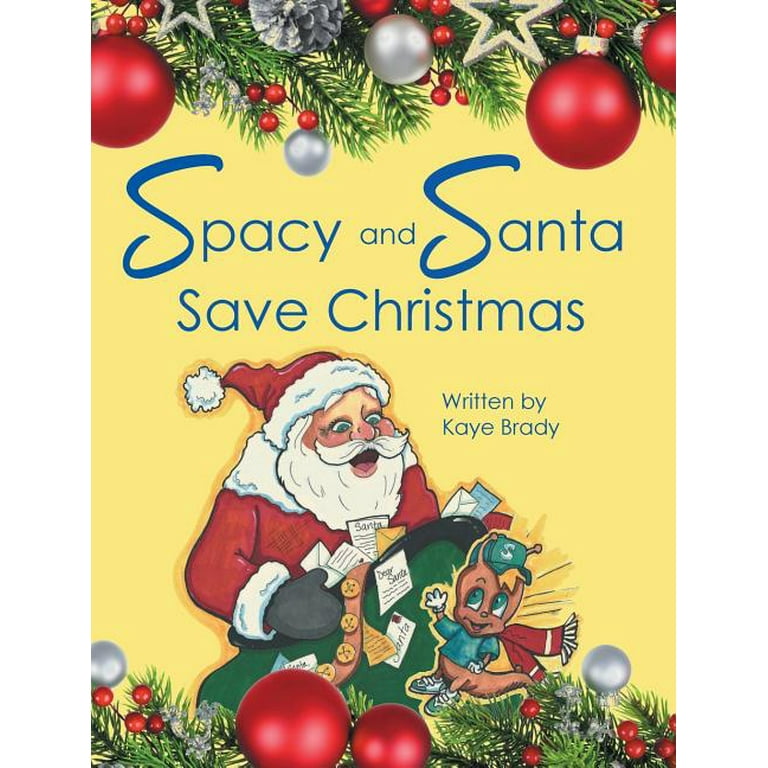The cover of this children's book prominently features a festive scene framed by Christmas tree branches and various ornaments. At the top of the vertical rectangular image, there is greenery adorned with red and silver bulbs, stars, and clusters of red berries. The background transitions to a pale yellow color where the title "Spacey and Santa Save Christmas" is written in blue font with large, curvy S letters beginning "Spacey" and "Santa." Below the title, it states "written by Kay Brady" in smaller text. 

The central part of the cover showcases a cheerful, cartoonish Santa Claus with his characteristic red hat, white beard, red jacket, and black mittens. Santa holds a large green pouch, presumably filled with letters and toys. Next to Santa, on his right, is Spacey, a little character with a round head, big green eyes, a kangaroo-like tail, two antennas, and a green hat with an "S" on it. Spacey is dressed in a blue shirt and a red scarf. 

Further embellishing the cover, more pine branches, silver and red ornaments, and red berries are found towards the bottom of the image, enhancing the festive atmosphere.